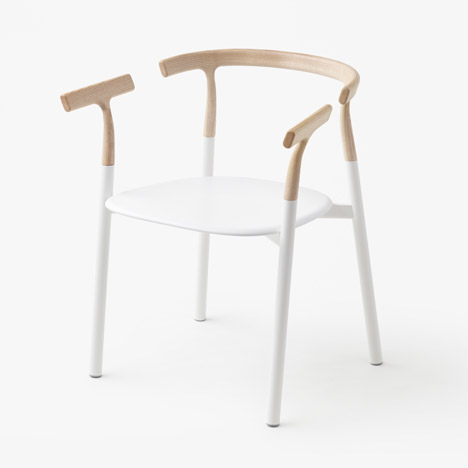The photograph showcases a distinctly modern, minimalist chair positioned against a stark white background and floor. The chair features a unique design with clean lines and a contrasting color scheme. Its bottom half, including the four legs and seat base, is a pristine white that may be metal or painted plastic, emphasizing its sleek, contemporary aesthetic. The top half of the chair, composed of the backrest and armrests, provides a natural contrast with its rich brown wood. The backrest is notably short, offering minimal support, and aligns with the wooden armrests, both crafted from the same material. A deliberate gap of about six inches separates the backrest from the armrests, giving the appearance of a cutout design element that adds to the chair's avant-garde style. The photograph's angle, showing the chair from a corner perspective, enhances the sense of depth and highlights its unconventional structure, making the chair seem almost like a stock image or an advertisement for modern furniture design.